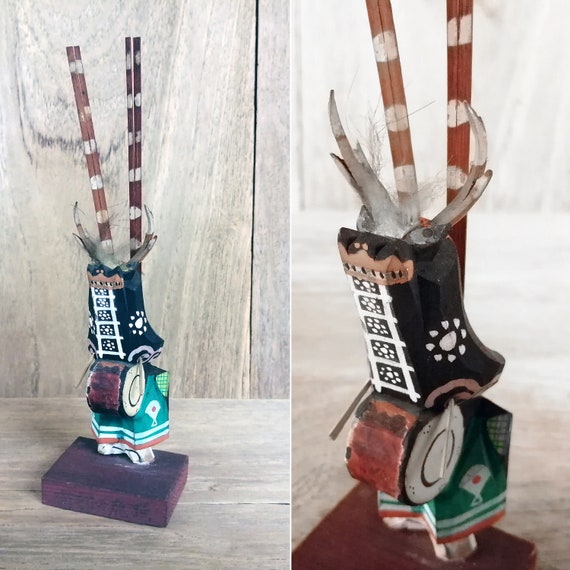The image features a two-part collage, with one photograph on the left and a zoomed-in version on the right, displaying a unique wooden decorative item placed on a light brown wooden surface. The background is a matching light brown wooden wall. The item depicts a character with a carved, cartoony deer-like head, complete with antlers, and is adorned in a black upper body and a green lower garment. The character is playing a drum positioned in front of it, using drumsticks held in both hands. The deer figure also features two horn-like structures on its head and two rod-like structures, resembling chopsticks, protruding from its back. The character stands on a square wooden block base. The paintwork includes detailed patterns in red, white, and black on the drum and the character’s attire. The photograph on the right offers a closer view, highlighting the intricate carvings and color details, suggesting slight variations in lighting or perspective rather than differing objects.